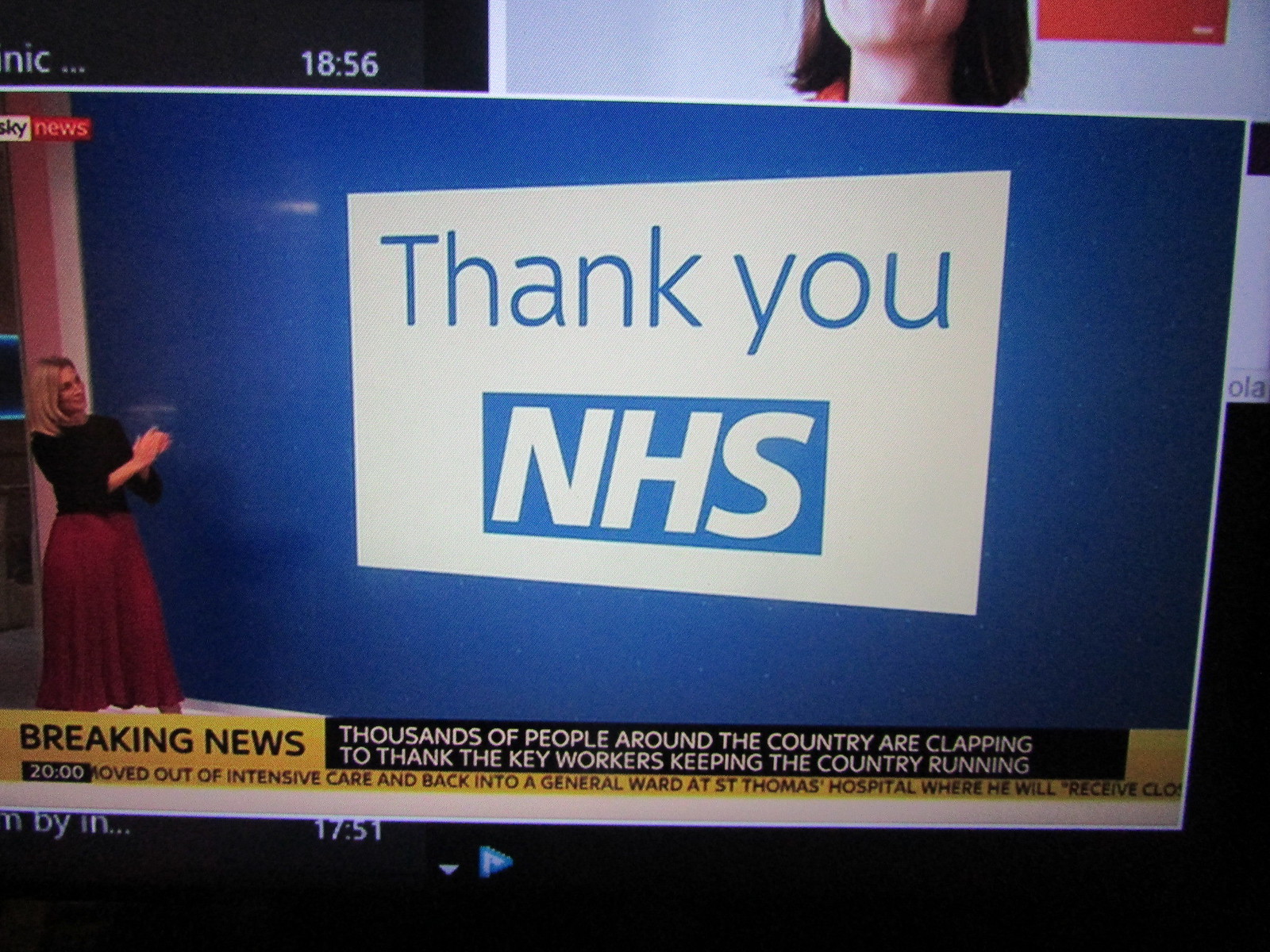The image depicts a television screen featuring a news broadcast from Sky News. Dominating the screen is a blue background with a white square prominently displaying the message "Thank You, NHS" in blue letters. To the left of this message stands a blonde, white female newscaster dressed in a black blouse and a long red skirt. She is clapping, echoing the sentiment expressed in the caption beneath her. The banner at the bottom, with white text on a black background, reads: "Thousands of people around the country are clapping to thank the key workers keeping the country running." Additionally, a yellow "Breaking News" banner mentions someone being moved out of intensive care and back into a general ward at St. Thomas Hospital, although the message is cut off. In the background, another screen shows a woman with short brown hair, and the numbers "1856" are visible. The image captures a moment of gratitude towards key workers amidst the ongoing news coverage.